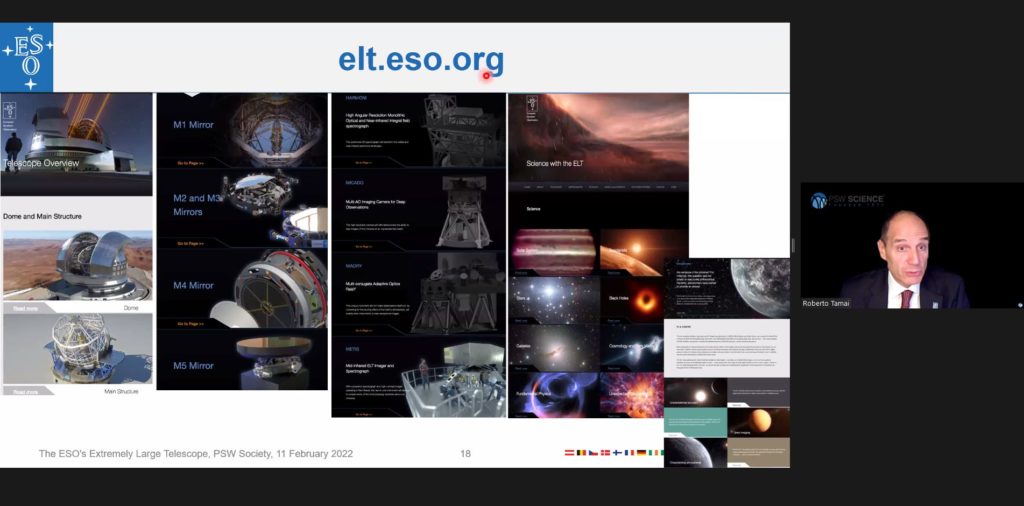The image appears to be a screenshot from a Zoom meeting or a presentation on a dark gray or black background. On the right side, there is a small video feed of a man named Roberto Tamai, who is dressed in a black suit, white shirt, and red tie. His name appears at the upper-left corner of his picture. 

The left side of the image features a presentation slide with the website address "elt.eso.org" displayed at the top in blue text on a white background. Below the address, the slide is organized into five columns of images related to telescopes and space equipment. The first column contains three images of technological devices, possibly related to outer space. The second column showcases images of cylindrical, drum-like objects. The third column displays various metallic items. The fourth column includes images of stars and planets. At the bottom of the slide, text reads, "The ESO's Extremely Large Telescope," followed by "PSW Society, 11 February 2022." Additionally, several small country flags, including Germany, are visible at the bottom right of the slide, though they are hard to identify. This comprehensive slide appears to be part of a broader discussion or presentation about the ESO's Extremely Large Telescope.